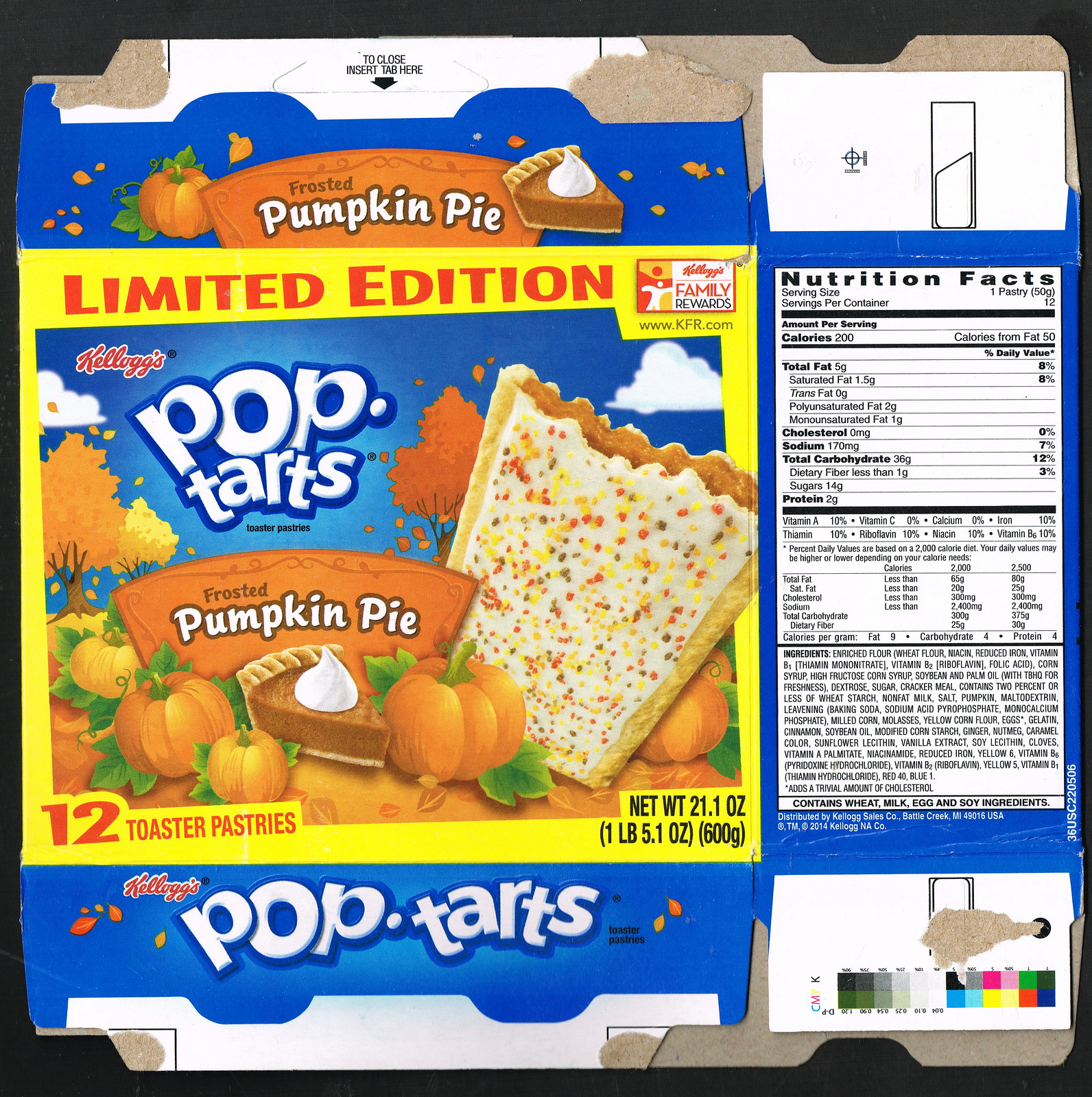This is an image of a flattened, real-life product packaging for limited edition Kellogg's Pop-Tarts in the Frosted Pumpkin Pie flavor. The front of the box features a vibrant blue background. In the center, there is a large, high-resolution image of a Pop-Tart with a partially bitten top, revealing the pumpkin pie filling inside. The Pop-Tart is frosted with white icing and adorned with festive red, yellow, and brown sprinkles.

Surrounding the Pop-Tart image are whimsical illustrations of orange pumpkins with green stems and leaves, emphasizing the seasonal theme. Below the Pop-Tart image, there is a depiction of a pumpkin pie topped with whipped cream, reinforcing the flavor variety. 

At the top left corner, the Kellogg's logo is prominently displayed in red. Just below the logo, a yellow banner with bold red letters announces that this is a "Limited Edition" product. The iconic Pop-Tarts logo, with its blue outline and white text, is positioned near the image of the pumpkin pie and the central Pop-Tart.

At the bottom of the packaging, it states "12 Toaster Pastries, Net Weight 21.1 oz (1 lb 5.1 oz) 600 g" to indicate the quantity and weight of the contents. 

Due to the flattened state of the carton, the tabs and part of the inside are visible, revealing the plain cardboard color and the print information. The right side of the image also shows the nutrition facts label with a white background and black text, detailing the serving size of one 50-gram pastry along with other nutritional information and an ingredient list.

This detailed visual presentation of the packaging provides a comprehensive understanding of the product, celebrating the limited edition Frosted Pumpkin Pie Pop-Tarts in a festive and informative manner.